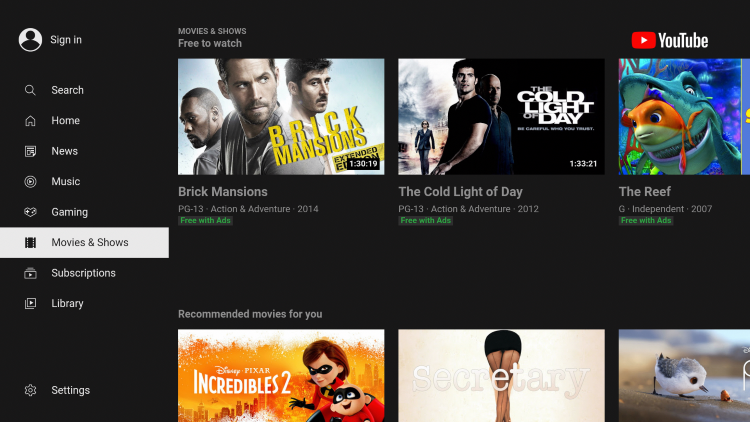The image depicts the YouTube website displayed in dark mode, characterized by a charcoal black background. The left side features a vertical menu starting from the top with a human silhouette icon labeled "Sign In." Below it are icons for "Search" (magnifying glass), "Home" (house), "News" (newspaper), "Music" (record), "Gaming" (game controller), and "Movies and Shows" (film strip), the latter of which is currently selected. Further down the menu are options for "Subscriptions," "Library," and "Settings."

In the upper right corner, the YouTube logo—a red rectangle with a white play button—stands out. Below the logo, there is a section titled "Movies and Shows Free to Watch," showcasing three titles: 

1. "Brick Mansions" (PG-13, Action and Adventure, 2014), available free with ads.
2. "The Cold Light of Day" (PG-13, Action and Adventure, 2012), available free with ads.
3. "The Reef" (G, Independent, 2007), available free with ads.